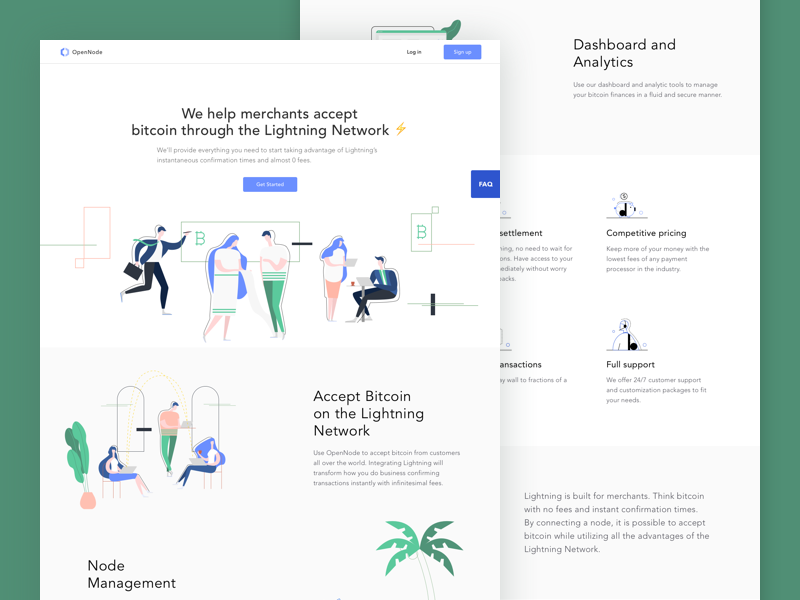Two overlapping infographic-style screen captures are presented against a mid-toned teal green background. Both windows feature a clean white background with blue logos at the top. The first window begins with a black header that reads "Log In" followed by a blue box. Below this, the text in black states, "We help merchants accept Bitcoin through the Lightning Network," accompanied by a small gold lightning bolt icon. Beneath this, two black text lines lead to a blue "Get Started" button. Illustrative graphics include a man wearing a blue jacket and black pants holding a briefcase, a woman in white with long blue hair, and a man dressed in white and green. The blue-haired woman and blue-jacketed man reappear, with the man now shown holding a laptop. A blue "FAQ" button is also present. Further down, the text "Accept Bitcoin on the Lightning Network" is displayed near a palm tree graphic and illustrations of the aforementioned characters sitting. The label "Node Management" appears in black text.

The second window, partly obscured by the first, features a black font on a white background. The header reads "Dashboard" and "Analytics," followed by two sentences in black text. Below, several icons are visible, although partially cut off by the first window. Three sections maintain clarity: the first with the header "Competitive Pricing" above a sentence or two, accompanied by a blue and black icon; the second with "Full Support" and a person icon in black, white, and blue, depicting someone wearing headphones, alongside the text "We offer 24-7 customer support and customization packages to fit your needs." The bottom of the window concludes with a statement in black text: "Lightning is built for merchants. Think Bitcoin with no fees and instant confirmation times. By connecting a node, it is possible to accept Bitcoin while utilizing all the advantages of the Lightning Network."